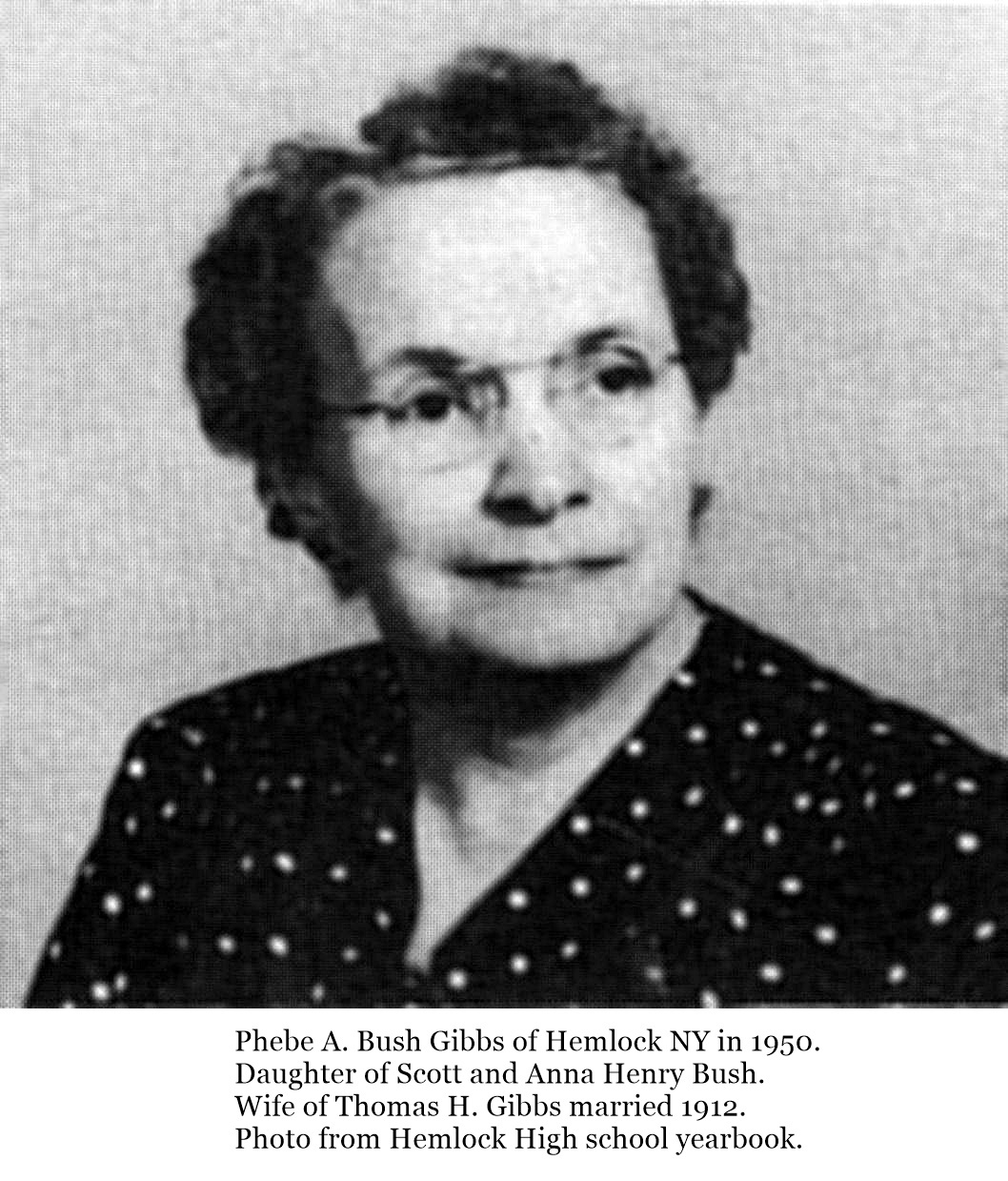This is a grainy, black and white photograph from the Hemlock High School yearbook, depicting Phoebe A. Bush Gibbs of Hemlock, New York, taken in 1950. The text footer reveals that Phoebe is the daughter of Scott and Anna Henry Bush, and wife of Thomas H. Gibbs, whom she married in 1912. Phoebe is shown wearing wire-rimmed glasses and a dark polka-dotted blouse with a V-neckline. Her hair is short and curly, and she appears to be half-smiling while looking slightly to the left. The background is a light gray shade, suggesting a formal yet softly lit setting. The image, while somewhat blurred and old, captures her composed and peaceful demeanor.